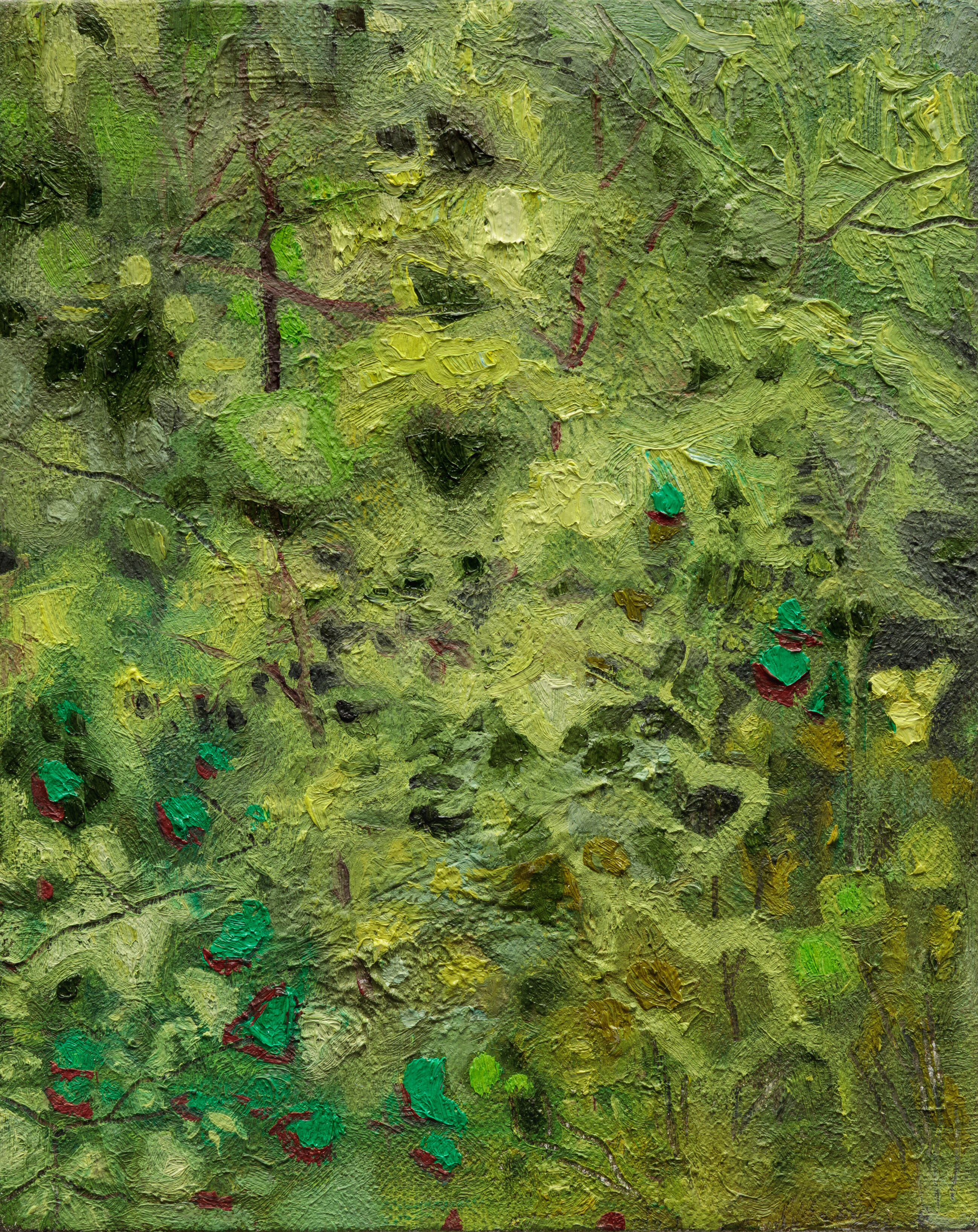This image is an impressionist painting depicting a forest with an emphasis on various shades of green and brown. The painting is textured, perhaps on a material resembling a checkered screen or some kind of wire mesh, which adds depth and complexity. The top part of the painting features tree trunks and branches, predominantly brown, extending from the corners and blending into a lighter green background. The bottom of the painting showcases darker, splotchy areas of green and brown, mimicking leaves and foliage. The central area is filled with multiple brush strokes and shades of green, creating the impression of dense woodland. Some areas of the background may be black or brown, adding a contrasting depth to the vibrant green shades. Overall, the painting captures the essence of a lush, densely wooded scene with a textured and layered feel.